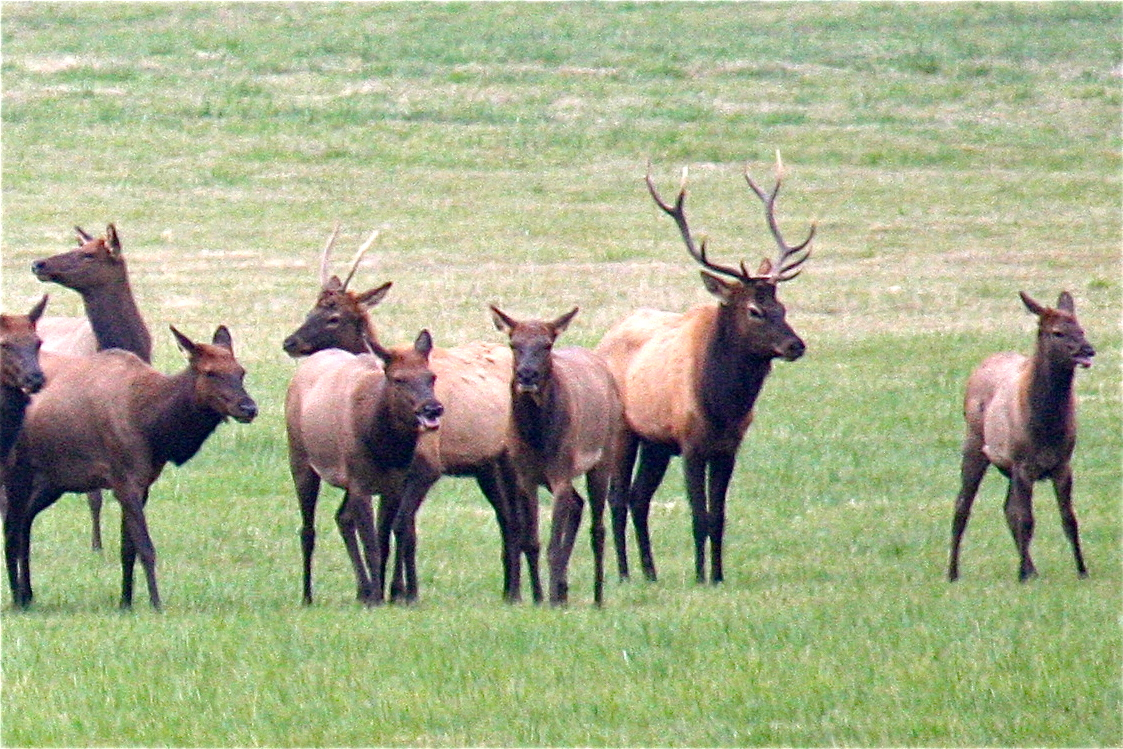A grainy, low-resolution photograph shows a herd of eight elk standing in a wide-open grassy field. The grass in the foreground is a bright green, though there are patches of light tan, indicating it is slightly dried but not entirely browned out. The elk, mostly facing toward the camera and slightly to the right, display a range of brown hues with darker shades on their faces, chests, and legs, and lighter tones on their backs. Two of the elk have antlers: one, positioned second from the right, boasts a large, elaborate set with many branches, while another, seated two places to the left, has small, straight antlers. The remaining elk, which appear to be a mix of females and juveniles, are without antlers. Some of the elk have their mouths open, exposing their pink tongues. No other elements are visible in the photograph beyond the expansive field of grass.